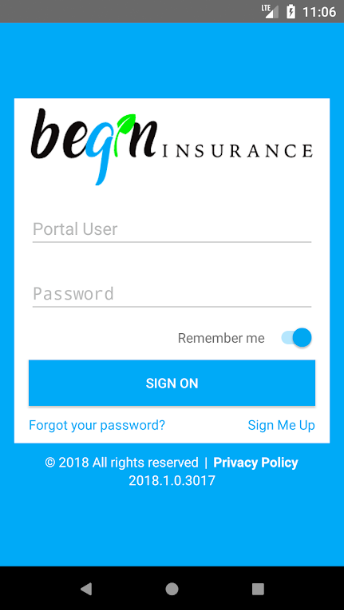The image depicts the login screen of a web application, captured from a tablet or smartphone, as indicated by the status icons in the top-right corner. The signal strength icon shows a bit over a third full in white, with the rest in dark gray, accompanied by an "LTE" label denoting 4G data connectivity. On the far right, a fully charged battery icon with a lightning bolt indicates that the device is plugged in but fully charged. Adjacent to these icons, the time "11:06" is displayed within a dark gray rectangle, though it is not specified whether it is AM or PM.

Below this, the screen transitions to a dark blue background and contains a central white rectangle. The top of this rectangle features the text "BEGIN" stylized in various colors and fonts: the letters "b," "e," and "n" are black, the "g" has a unique curled design and is blue, and the "i" is represented by a green leaf. Beneath this is the word "INSURANCE" in black text. Further down, the fields for "PORTAL USER" and "PASSWORD" are displayed, accompanied by a "REMEMBER ME" checkbox that is checked, indicating a blue toggle slider in the active position. 

At the bottom right, there is a blue button with white text that reads "SIGN ON." To the lower left of this button, in blue text, are the options "FORGOT YOUR PASSWORD?" and "SIGN ME UP." Within the blue area of the background, the screen also includes copyright information in white text: a copyright symbol (©), "2018 ALL RIGHTS RESERVED," a vertical line, and the term "PRIVACY POLICY" in bold white. The version number "2018.1.0.3017" is centered below this information.

Below these elements, a black bezel marks the bottom of the device, featuring navigation icons: a gray arrow for going back, a circle for minimizing the window, and a rectangle for maximizing it.